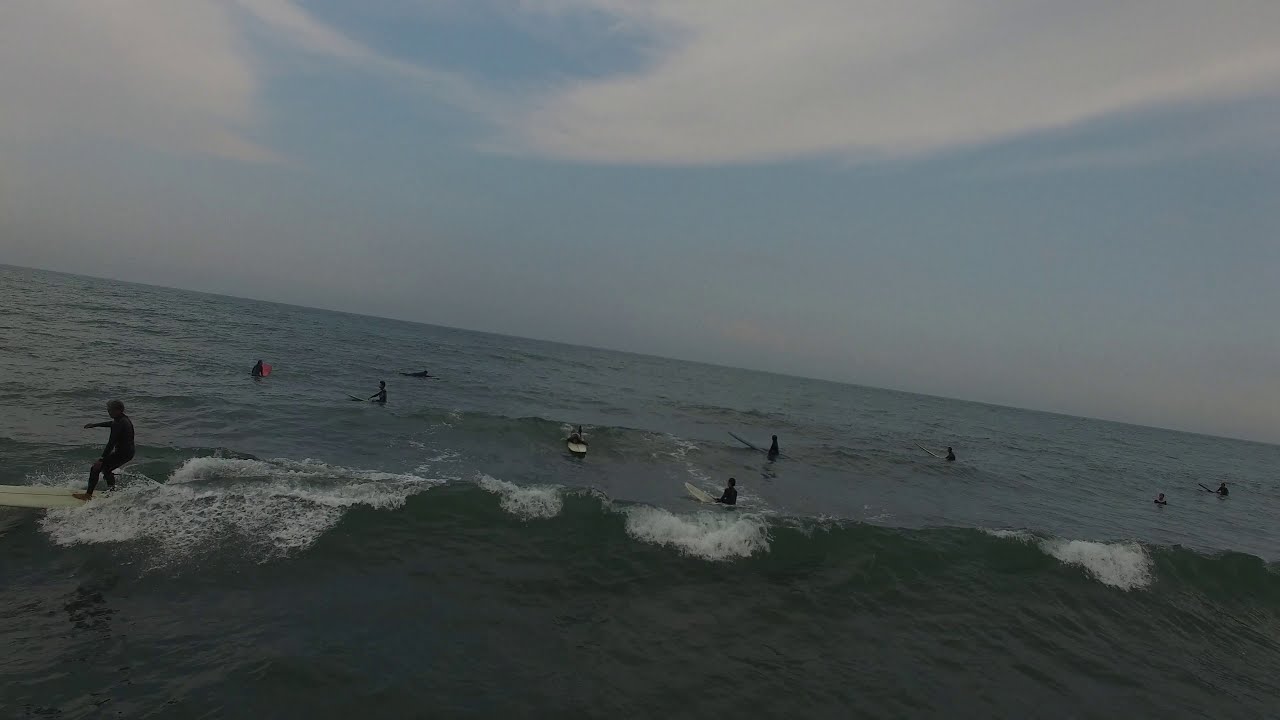This photograph captures a dynamic shoreline scene where a group of roughly ten surfers interact with modest waves on an overcast day. The image, slightly underexposed, highlights two distinct sets of waves. In the foreground, a surfer on a longboard rides a two to three-foot wave, moving toward the left side of the frame. Behind him, another longboarder is in the process of standing up on a new wave. The rest of the surfers, scattered throughout the lower half of the photo, either sit or lay on their boards, awaiting their turn. The water varies from dark tones in the foreground to a grayer hue further back, complemented by white foamy caps atop the waves. Above, the sky is a mix of blue with wispy, white clouds, filling the upper portion of the image. Despite the somewhat gloomy atmosphere, the scene conveys a tranquil yet invigorating moment as the surfers engage with the gentle, rolling waves.